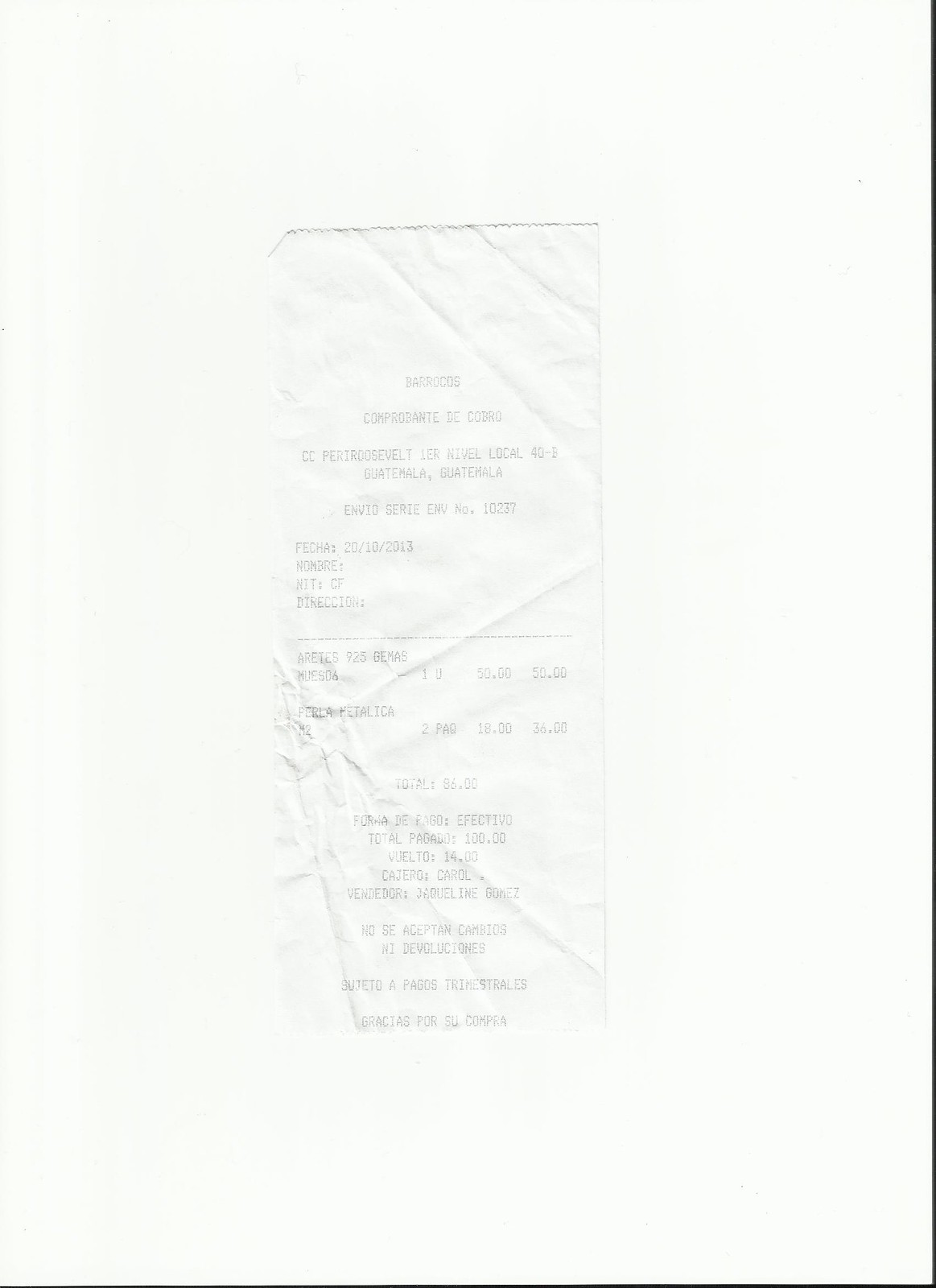This image depicts a highly faded and crinkled receipt, likely a testament to its age and having been carried in someone's pocket for an extended period. The receipt, which seems to originate from an auto parts store, details the purchase of a single item priced at approximately $6. Unfortunately, the text is obscured to the point of being illegible, even when magnified. The purchase date is discernible as February 10th, 2013. Adding to the difficulty of interpretation, the receipt is photographed against a white background, blending into it and further complicating any attempts to read the already faded print. The reason for capturing this image remains unclear.